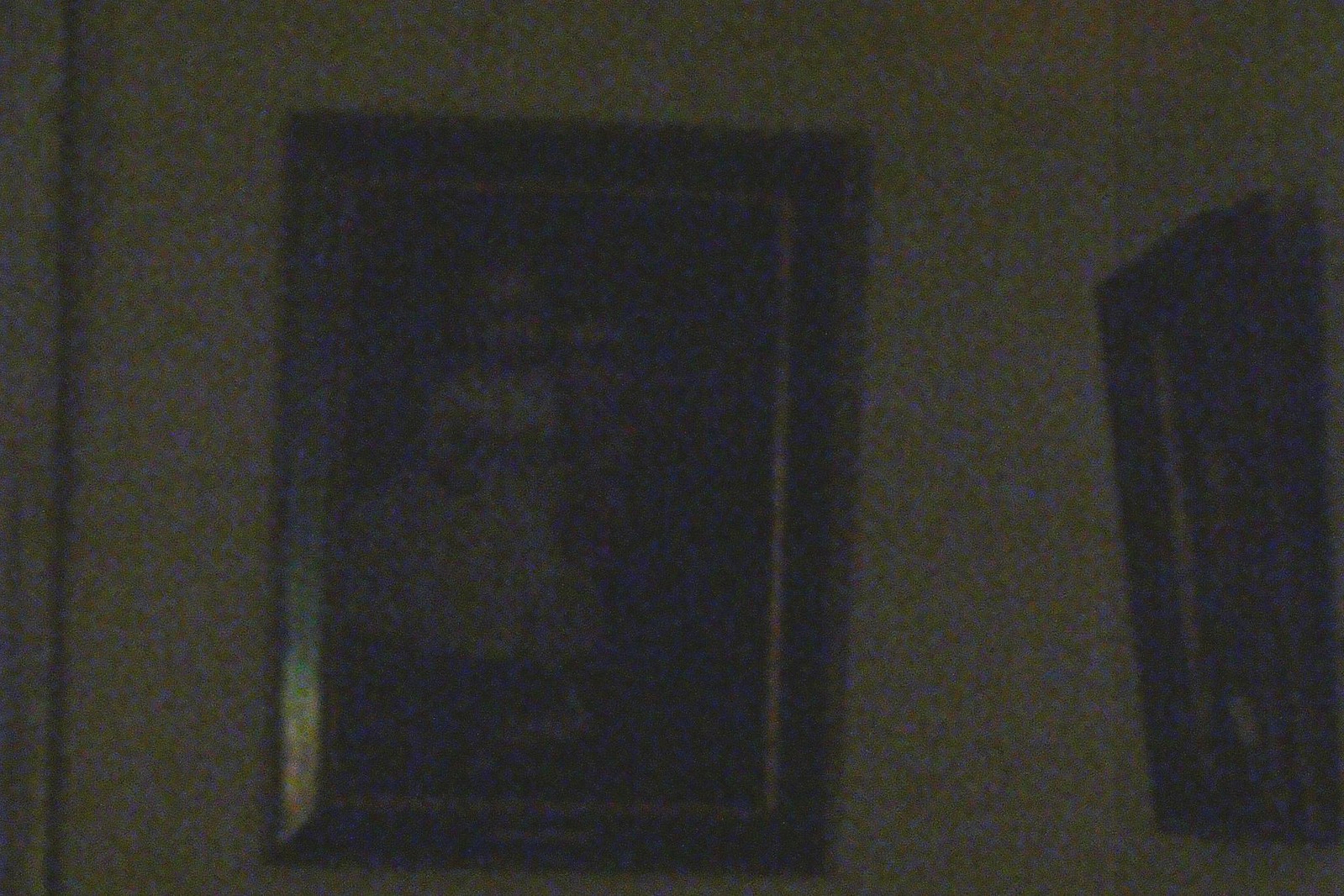In this dimly lit and blurry image, it's challenging to discern the exact setting or subjects. It appears to be captured in an art museum or hallway, characterized by framed artwork on the walls. Dominating the center is a framed photograph featuring a child in what seems to be a christening dress, framed with a dark outer frame and a distinct silver inner border. Off to the right, another framed piece is visible, set slightly askew towards the wall. Despite the poor lighting and heavy pixelation, a black vertical line on the far left likely outlines a doorframe, running from the top to the bottom of the image and intersecting it about a quarter of an inch in. The overall ambiance suggests a quiet, possibly historical environment, though details remain indistinguishable due to the image quality.